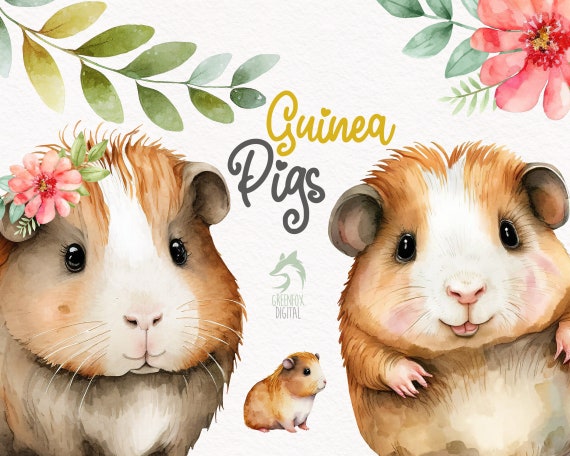This postcard features a charming, watercolor illustration of three adorable, cartoonish guinea pigs. Dominating the foreground are two large guinea pigs, with a smaller one situated towards the background, giving the appearance of depth. The guinea pig on the left, likely a female, is adorned with a pink flower and green leaves on its head, adding a delightful touch of personality. The one on the right, presumably a male, is depicted with an endearing open-mouthed smile, revealing a tiny tongue. The smaller guinea pig in the center, likely further back due to perspective, sits lower and looks to the right.

The background of the postcard is a simple white, akin to a blank wallpaper, ensuring the guinea pigs stand out vividly. Adorning the top of the postcard are additional floral elements: a leafy stem above the left guinea pig and a pink flower with green and blue leaves above the right. Centrally positioned in elegant cursive is the label "guinea pigs," accompanied by the logo for Green Fox Digital, featuring a green fox in profile. This whimsical and detailed artwork makes for a delightful and inviting front cover for a gift card or postcard.